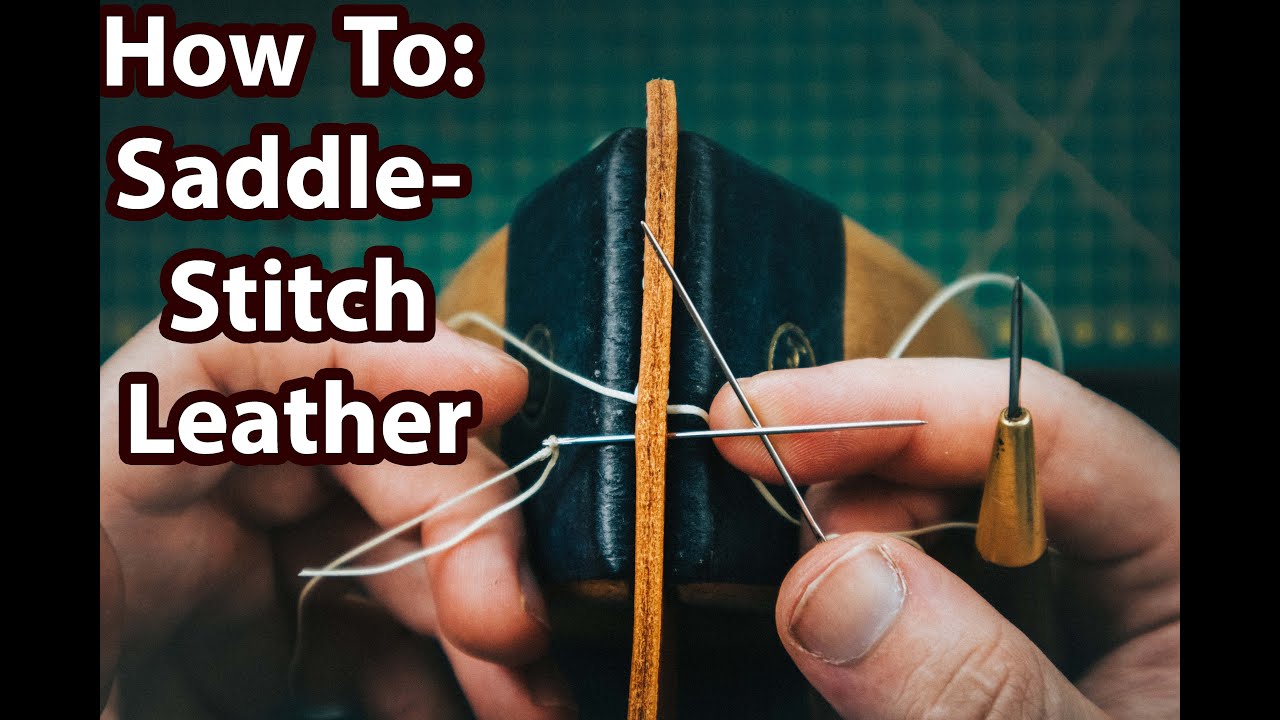The image, a title frame likely from a blog or vlog, showcases a step-by-step guide on "How to Saddle Stitch Leather." Framed by thick vertical black borders on both the left and right sides, the centerpiece features a close-up of a leatherwork project. A large brown piece of leather dominates the middle of the picture, almost reaching the top, flanked by additional swatches of blue and brown fabric. At the bottom center, a needle with white thread is being inserted into the leather from left to right, still partially visible on the left side of the leather. The right hand, holding another needle, appears on the lower right, with the thumb extending beyond the frame, while the left hand, displaying the forefinger, middle finger, and ring finger, extends off the lower left corner of the image. A notable detail on the right forefinger is a tool with a brown rounded bottom and a gray top, threaded with some material. The background hints at a green surface with yellow dots. The text "How to Saddle Stitch Leather" appears prominently on the left side in bold white letters with a brown outline, serving as a clear instructional label for the image.